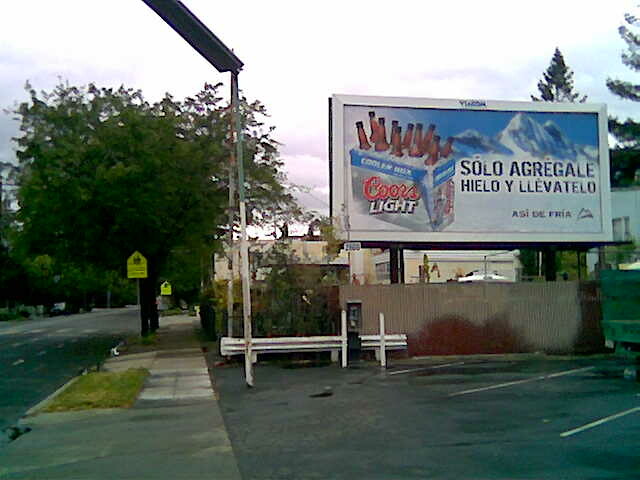In this detailed neighborhood scene, you can see a small local store amidst a quaint residential area. The sky is predominantly overcast with a slight hint of blue peeking through. A towering tree, lush with green foliage, dominates the foreground. The street is a three-lane passage lined with numerous trees, providing a green canopy along the sidewalk. Adjacent to the street, a driveway extends into a modest parking lot bordered by a metal fence.

A vintage payphone, affixed to a pole, stands as a relic of the past. A prominent white sign with a blue background featuring white mountains advertises Coors Light, with an image showcasing bottles poking out from a package. Several marked parking spaces are visible in the parking lot next to a concrete wall and a green dumpster, completing the everyday charm of this neighborhood corner.